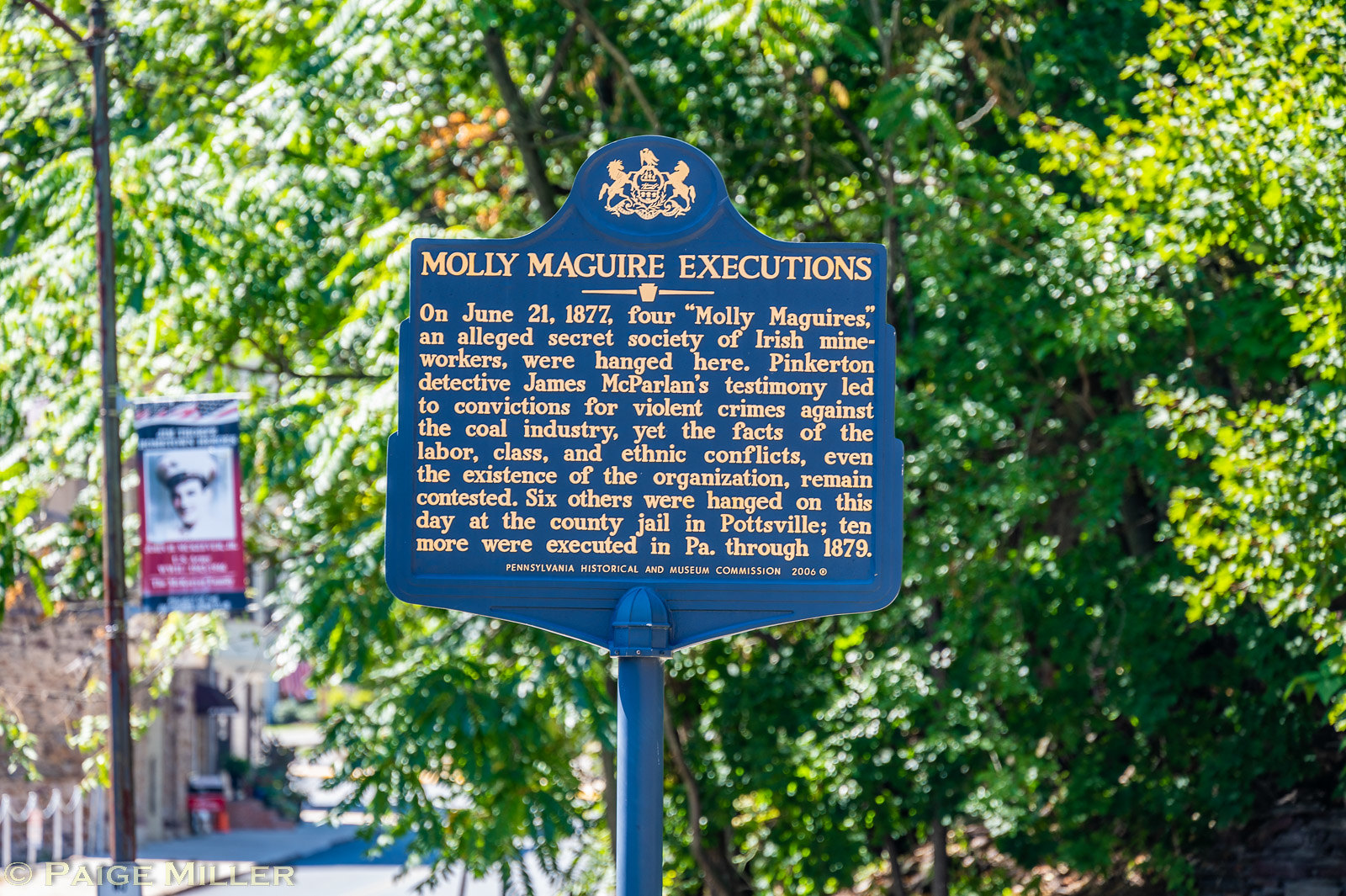The photograph depicts a heavily-treed area, possibly a park or visitor center, with a dense backdrop of green-leaved trees. To the left, near the bottom, there's a partially visible sidewalk. In front of what could be a visitor center, there's a wooden post displaying a red, white, and blue banner featuring a blurred image of a man in military attire, with American flags at the top. Centered in the image's foreground is a prominent blue metal sign on a vertical post, adorned with a crest at the top, flanked by two golden lions. The sign's header reads "Molly Maguire Executions" in gold text. Below, it details that on June 21, 1877, four members of the alleged secret society of Irish mine workers, the Molly Maguires, were hanged based on the testimony of Pinkerton Detective James McParland, who secured convictions for violent crimes against the coal industry. Despite these convictions, disputes about labor, class, and ethnic conflicts, and even the group's existence, persist. Additionally, six others were executed at the county jail in Pottsville that same day, with ten more executions occurring in Pennsylvania through 1879. Below the main paragraph is a small, unreadable line of text.